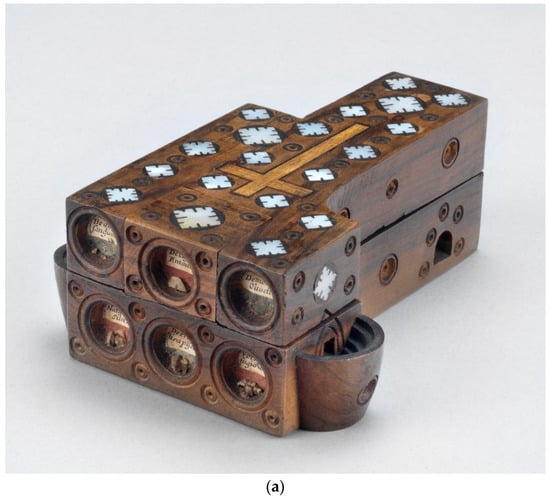This image showcases a meticulously designed wooden box, likely of religious significance, prominently displaying a gold cross etched into its top surface. The box is crafted from dark wood and adorned with intricate white designs and symbols, including what may be light blue snowflakes or clovers. Its detailed construction reveals multiple interlocking parts, with notable features such as two rows of circular cutouts on the front, each row containing three circles. Some of these circles contain small, partially readable text including letters like G-I, D-E, and M. The side of this box features a protruding, pot-like structure, which may serve for holding or dispensing liquid or other items, hinting at a function related to religious sacraments like communion. The entire piece is set against a white background, indicating it could be one image in a series, and is labeled with an "A" in brackets, suggesting it is part of a larger collection.